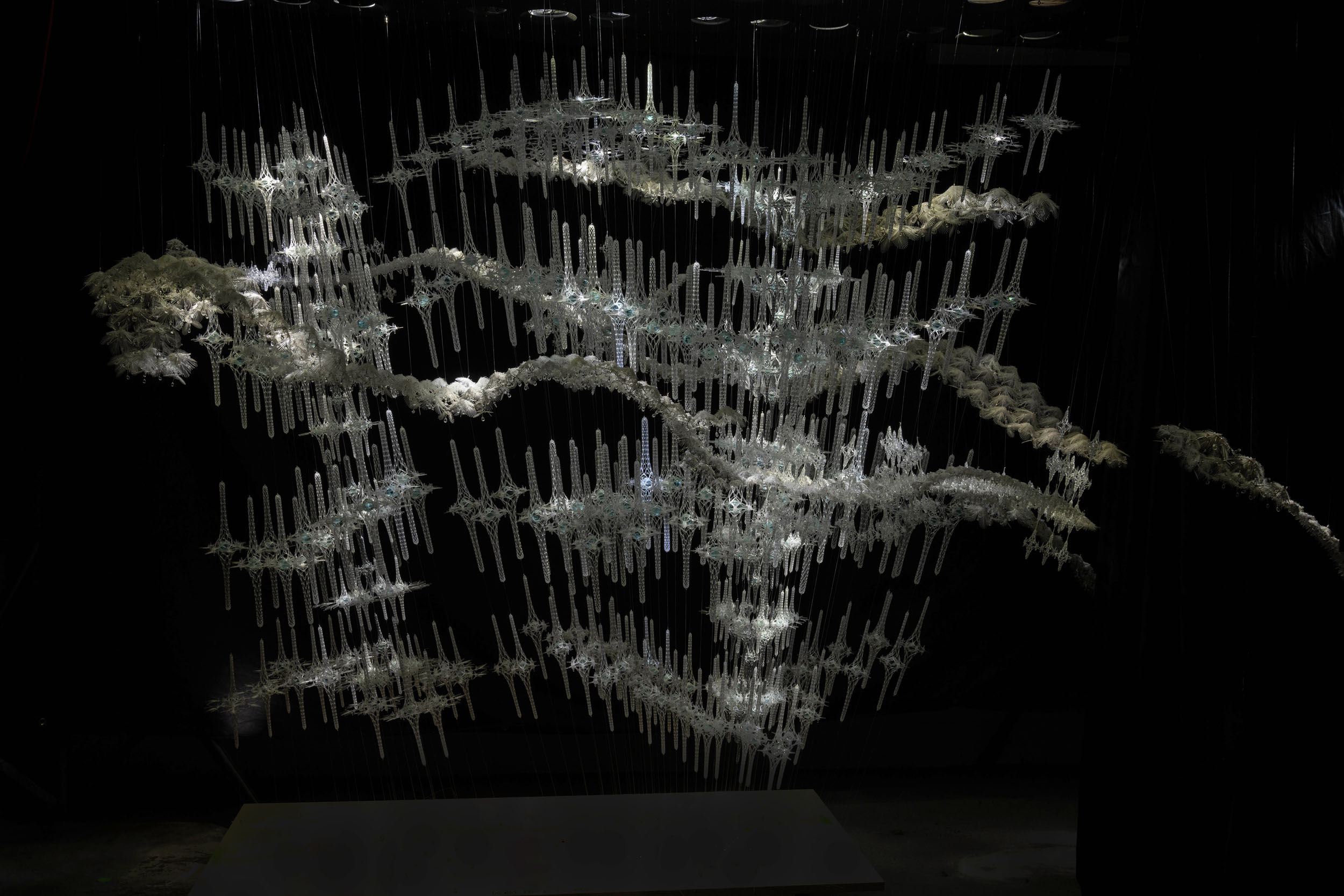The image depicts a captivating 3D art installation set against an entirely black, opaque background. Suspended from the ceiling by wires, the installation features a multitude of translucent, star-shaped structures arranged in an abstract, cityscape-like formation. The central element is a long post, from which numerous white or gray, almost syringe-like shapes extend outward, creating an intricate array of compressed diamond forms. These structures appear to form a surreal, undulating landscape reminiscent of mountains or waves. The overall effect is both mesmerizing and eerie, with the translucent elements lending an otherworldly, almost ethereal quality to the installation.